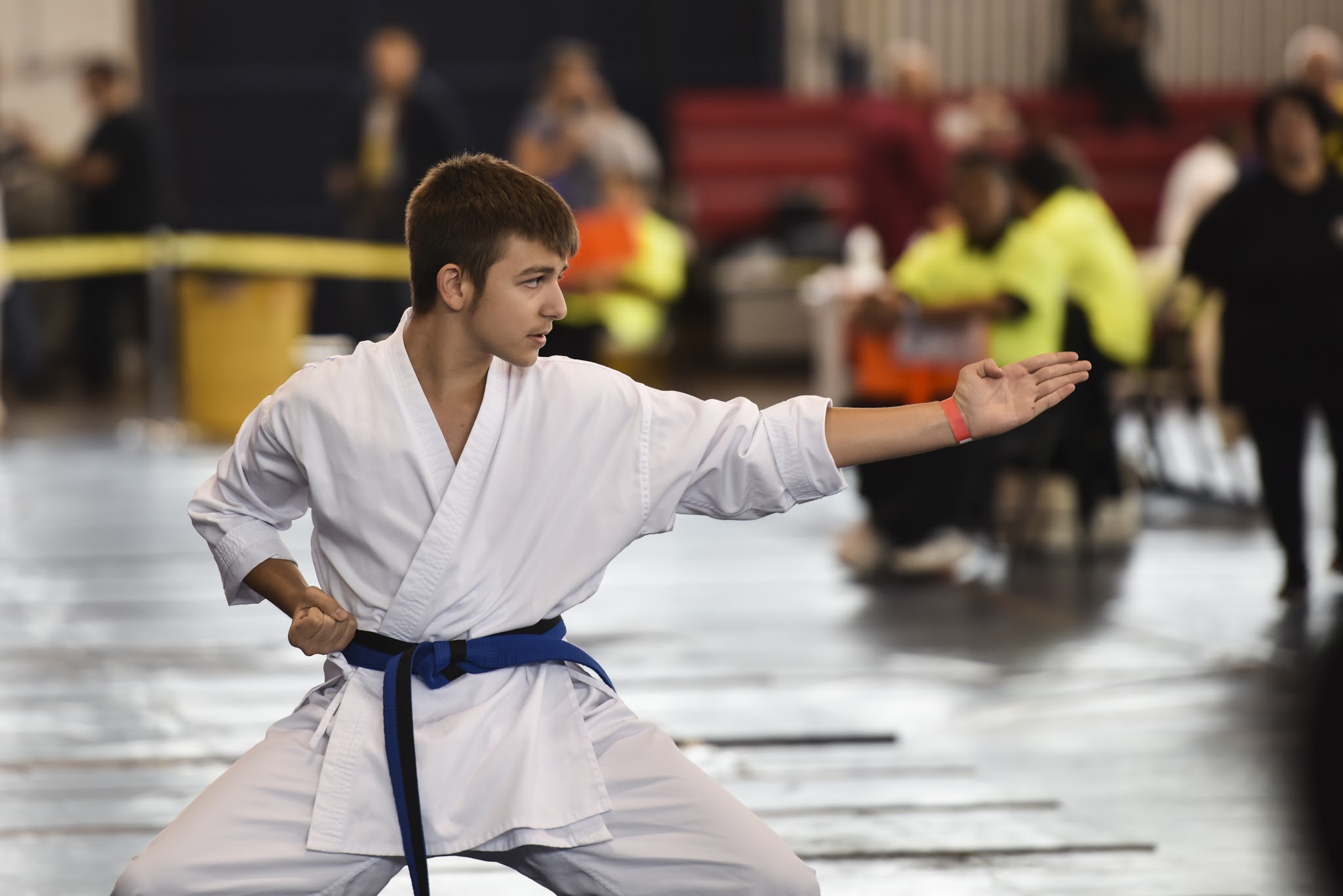This is a color photograph capturing a young boy engaged in a martial arts stance, likely either karate or taekwondo. Positioned centrally and shown in profile, he faces to the right. The boy has short brown hair and is slightly crouched down, giving emphasis to his athletic posture. His right arm is pulled in towards his torso with a closed fist, while his left arm is outstretched to the side, hand open with fingers closely grouped together. He is dressed in the traditional white martial arts uniform, cinched at the waist with a dark blue belt adorned with a black stripe. An orange bracelet or watch is visible on his wrist. The scene is set on a black mat that reflects the room's lighting, adding a subtle shine. The background is blurred, filled with spectators who are standing or seated, possibly on red bleachers, observing the action. The overall focus remains firmly on the young boy's disciplined form.